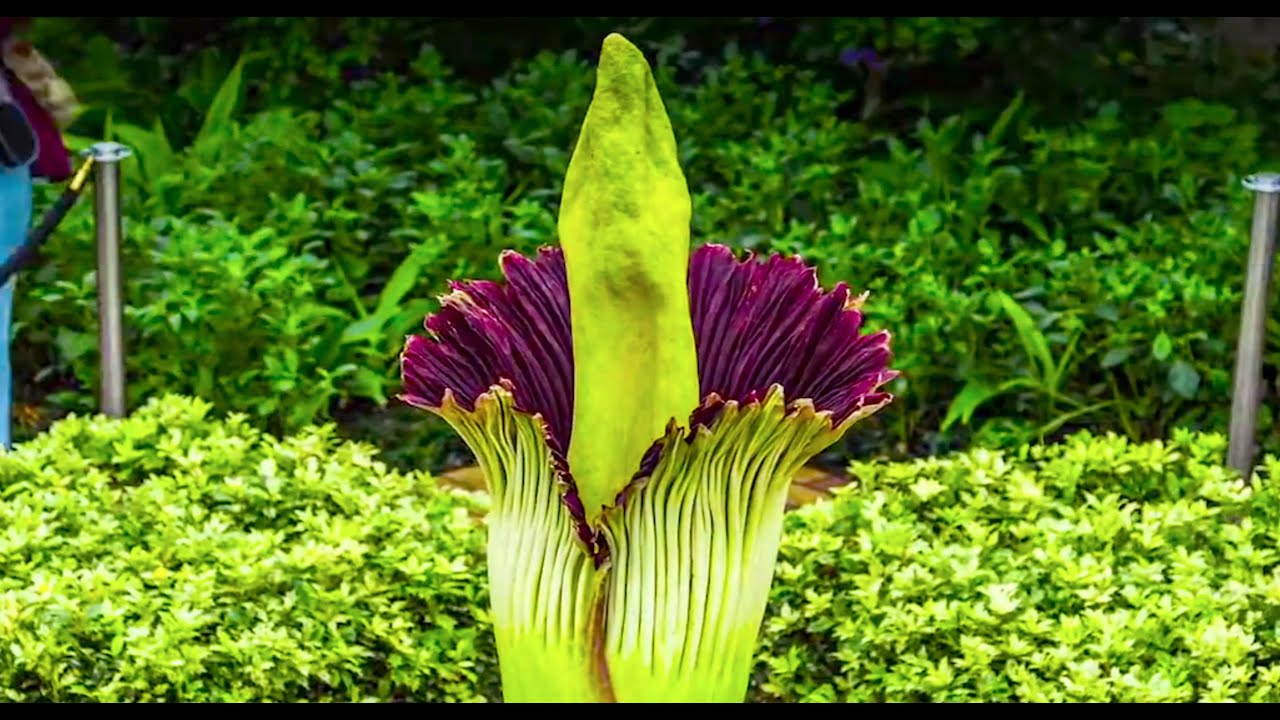The photograph captures a striking and unique botanical spectacle: the corpse flower, showcased in the center of a garden or arboretum. This immense plant features a towering, neon green stalk that protrudes from the middle of a large, chalice-shaped bloom. The interior of this bloom reveals a deep purple hue, contrasting vividly with the mint-green central section. Surrounding the focal plant, the backdrop includes a variety of green tones, from the black and deep green of distant foliage to the light yellow-green of smaller, adjacent bushes. Adding to the scene of contemplative display, metal posts and a felt rope cordon off the area around the corpse flower, suggesting a formal exhibition setup. Despite the absence of actual visitors in the shot, the setup implies a space curated for public admiration on what appears to be a gloomy day.